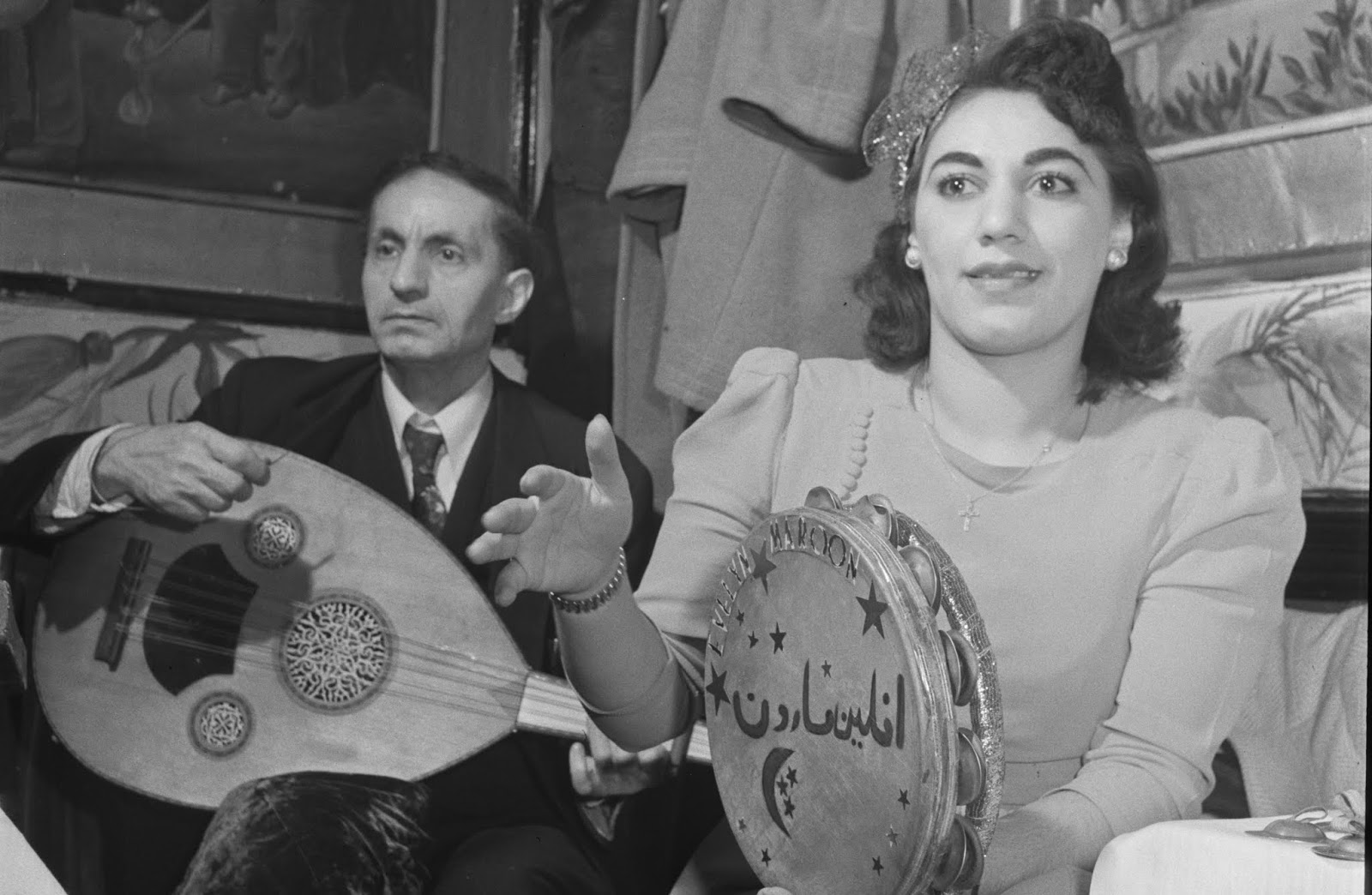This black and white photograph captures an older gentleman and a younger woman, both poised with musical instruments. The man, possibly in his fifties or sixties, is seated on the left. He wears a suit and tie and clutches a banjo-like instrument with a rounded, geometric design, potentially a sitar. His slightly startled expression is framed by his dark hair. Behind him hangs a framed painting.

Seated next to him is a woman in her thirties with shoulder-length dark hair adorned with a bow. Her dark eyes and bemused smile give her a puzzled yet charming appearance. She wears a dress, a cross necklace, earrings, and a bracelet or watch on her raised left hand. Her other hand rests on a tambourine, which features star and moon designs along with writing that appears to be in Arabic, hinting at "Evelyn Maroon." Behind her, a coat is draped over a chair. Both individuals share the spotlight in an intimate setting, creating a timeless scene of musical contemplation.